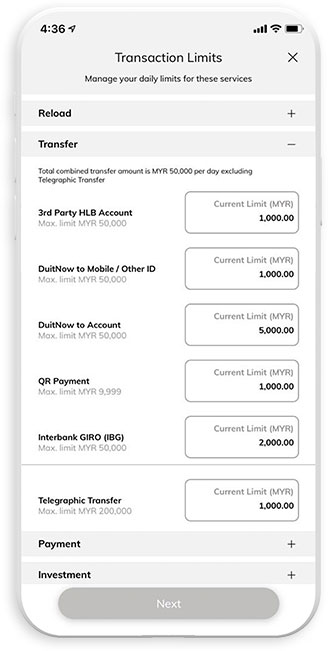Here's an optimized and detailed caption:

---

This screenshot captures a detailed interface from a smartphone application designed to manage transaction limits. The interface has a rounded rectangular border, shaded in gray. On the upper left corner, there's an arrow icon labeled with "436." Adjacent to this, the time and status symbols for Wi-Fi and battery usage are displayed. Centered at the top is a bold title "Transaction Limits" in black, followed by a gray 'X' icon to the right. Below the title is a smaller description, "Manage your daily limits for these services."

The main content is divided into several sections:

1. **Reload and Transfer:** The reload section is annotated with a plus symbol (+) and the transfer section with a minus symbol (−).
2. **Transaction Categories:** The categories listed, including "Third-party HLB Account," "Do it now to mobile/other ID," and "Do it now to account," have their respective descriptions in smaller, gray text.
3. **Limits and Amounts:** 
     - Next to each category on the left, labels show "Current Limit MYR" with accompanying limits displayed from top to bottom in bold black: MYR 1,000, MYR 1,000, MYR 5,000, MYR 1,000, MYR 2,000, MYR 1,000.
4. **Additional Categories:** 
     - Separate sections include "Telegraphic Transfer," which lists a maximum limit of MYR 200,000 and a current limit of MYR 1,000.
     - The "Payment" and "Investment" sections are each accompanied by respective plus icons (+).
5. **Action Button:** At the bottom of the screen, a gray elongated 'Next' button stands out, with the text in white.

This image provides a comprehensive view of the application’s functionalities for managing diverse transaction limits and financial activities.

--- 

This formatted description provides a clear and detailed overview of the screenshot, capturing all key elements and their arrangements.